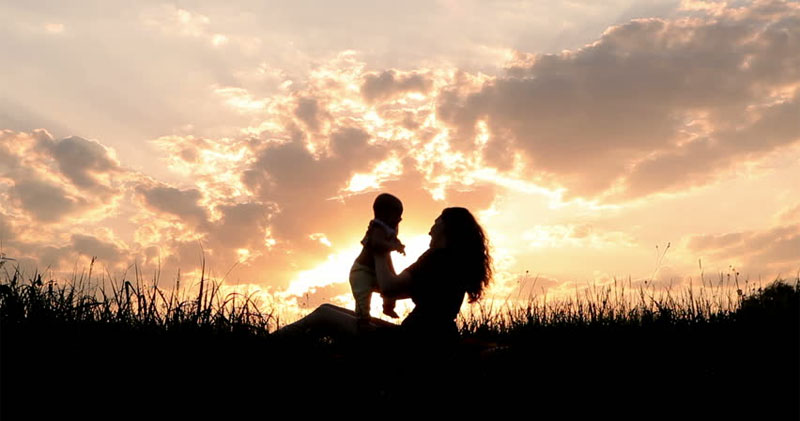Against the backdrop of a vibrant sunset, the silhouette of a mom with long hair and her toddler creates a captivating scene in an open country field. The mom, seated and facing left, tenderly holds up her baby in her arms, who faces her to the right. The foreground features a horizontal expanse of grass, adding to the rustic charm. The sky is a stunning display of colors, transitioning from a purplish hue at the top to a warm orange near the horizon. The setting sun casts a yellowish glow, illuminating the myriad of clouds in shades of purplish lavender, pink, and orange. The artistic backlighting enhances the silhouettes, highlighting the tender moment against the beautiful, fiery sky.